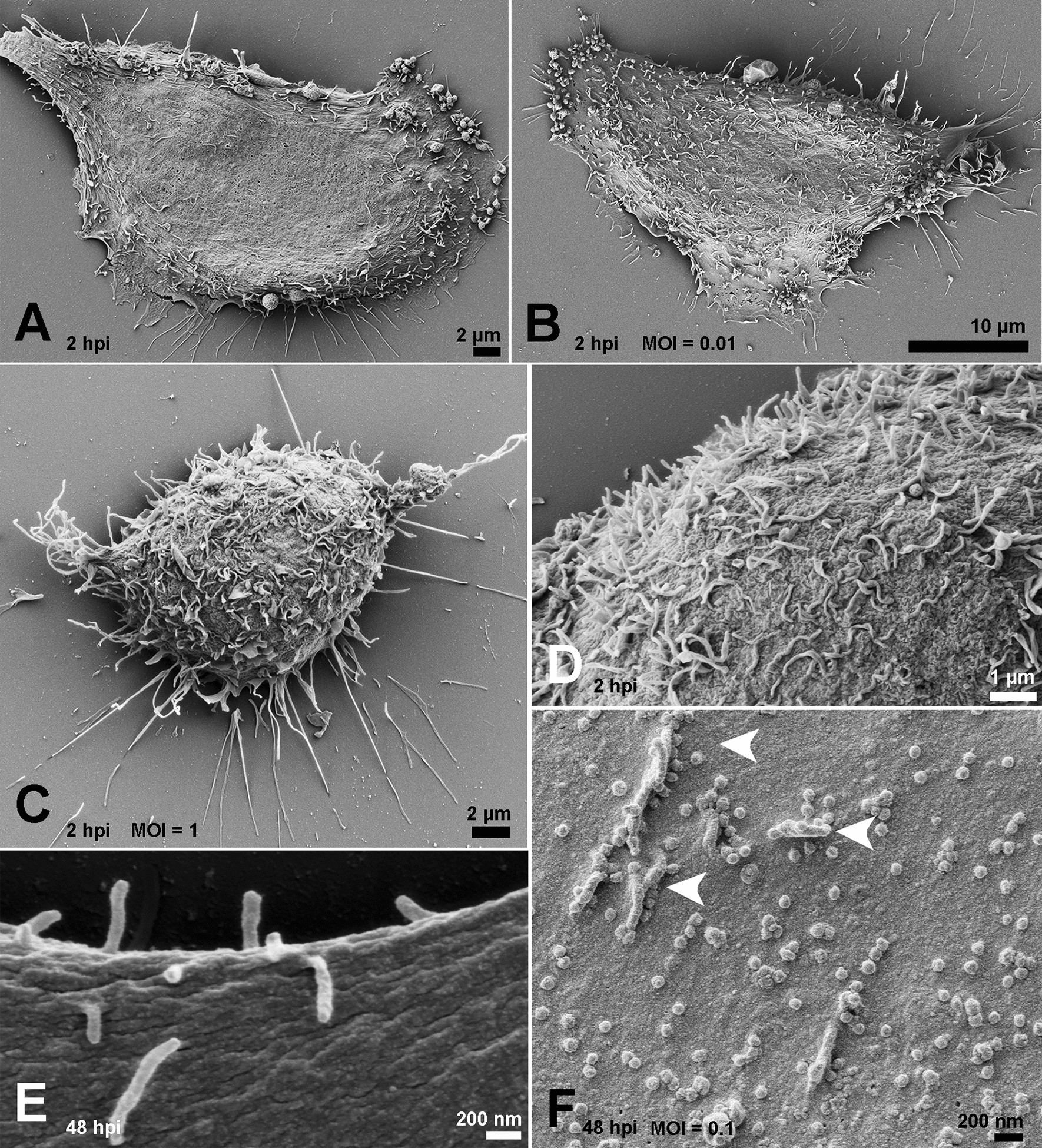This composite image features six detailed black-and-white microscopic photos labeled A through F, showcasing various stages of bacterial or mold development with distinct morphological characteristics and scales. 

- **Image A** (2 HPI, 2 micrometers): Displays an oblong, island-like structure with rough edges and hair-like protrusions on one side.
- **Image B** (2 HPI, MOI=0.01, 10 micrometers): Features an upside-down taco-like form covered in dots and elongated projections, more zoomed out than A.
- **Image C** (2 HPI, MOI=1, 2 micrometers): Shows a cylindrical shape with dense hairs, resembling a potato or heart.
- **Image D** (2 HPI, 1 micrometer): A close-up of a hairy surface, possibly a zoomed-in view of the structure in C.
- **Image E** (48 HPI, 200 nanometers): A highly detailed cross-section with visible worm-like structures, suggesting advanced growth stages.
- **Image F** (48 HPI, MOI=0.1, 200 nanometers): Features three arrows pointing to squiggly entities on a textured surface, indicating detailed formations at a high magnification.

These images collectively provide a sequential view of bacterial or mold growth, showcasing changes in structure and complexity at different time points and magnifications.